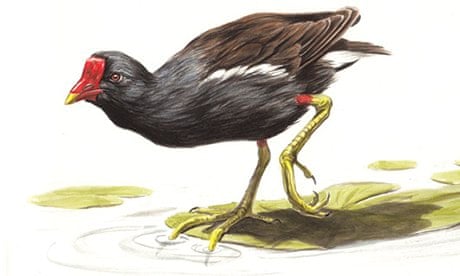This is a detailed drawing of a bird standing on a large yellow leaf, surrounded by smaller leaves and swampy puddles. The bird has a striking appearance with a black head and fine black feathers that cover its body up to its legs. It sports a red beak with the tip transitioning to yellow and a prominent red marking extending from its forehead to just above the beak. The edges of its wings exhibit a white line, while its rear features a distinct brown color. The bird's legs and feet are pale yellow, with a hint of red on top of the legs. One leg is raised with its talons touching the water, creating ripples. The bird appears to be walking westward, presenting an intricate and vibrant scene upon a white background.